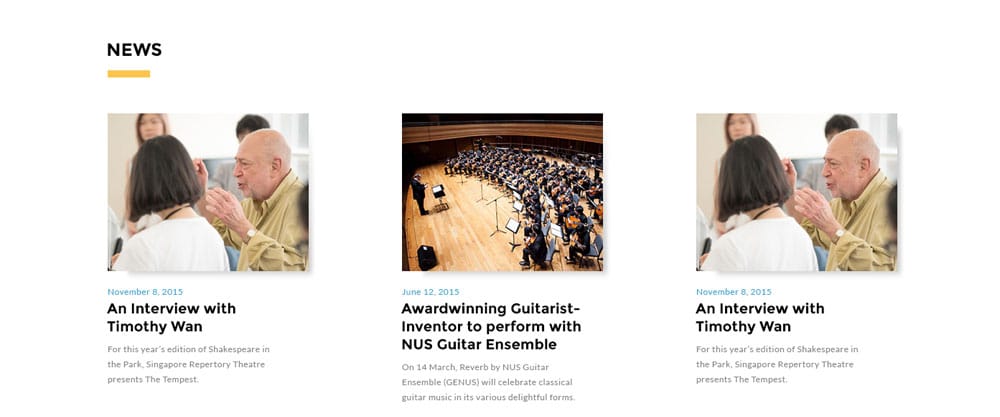A screenshot from a website reminiscent of Reuters, characterized by a specific coloration and font style, displays a NEWS section in bold capital letters. Below the NEWS header is a small yellow bar, followed by three images, two of which are identical.

The first image on the left is a profile picture of an older man with his hands raised, as if in mid-gesture. Although his mouth is not open, his expressive posture suggests he is speaking. Beside him is the back of a person, presumed to be a woman due to her attire, body shape, and shoulder-length brown hair. In the background, two blurred figures, one likely male and the other possibly female, are faintly visible.

Both the left and right images feature this same scene and are labeled as "An interview with Timothy Wan," with the date November 8, 2015, below. Accompanying text under this heading reads, "For this year's edition of Shakespeare in the Park, Singapore Repertory Theatre presents The Tempest."

The central image portrays a musical ensemble, possibly a symphony or orchestra, and is captioned, "Award-winning guitarist-inventor to perform with NUS Guitar Ensemble," dated June 12, 2015. Below this, the description elaborates, "On the 14th of March, reverb by NUS Guitar Ensemble will celebrate classical guitar music in various delightful forms."

Detailed and finely punctuated, this caption aims to provide a clear and descriptive understanding of the contents and context of the screenshot.